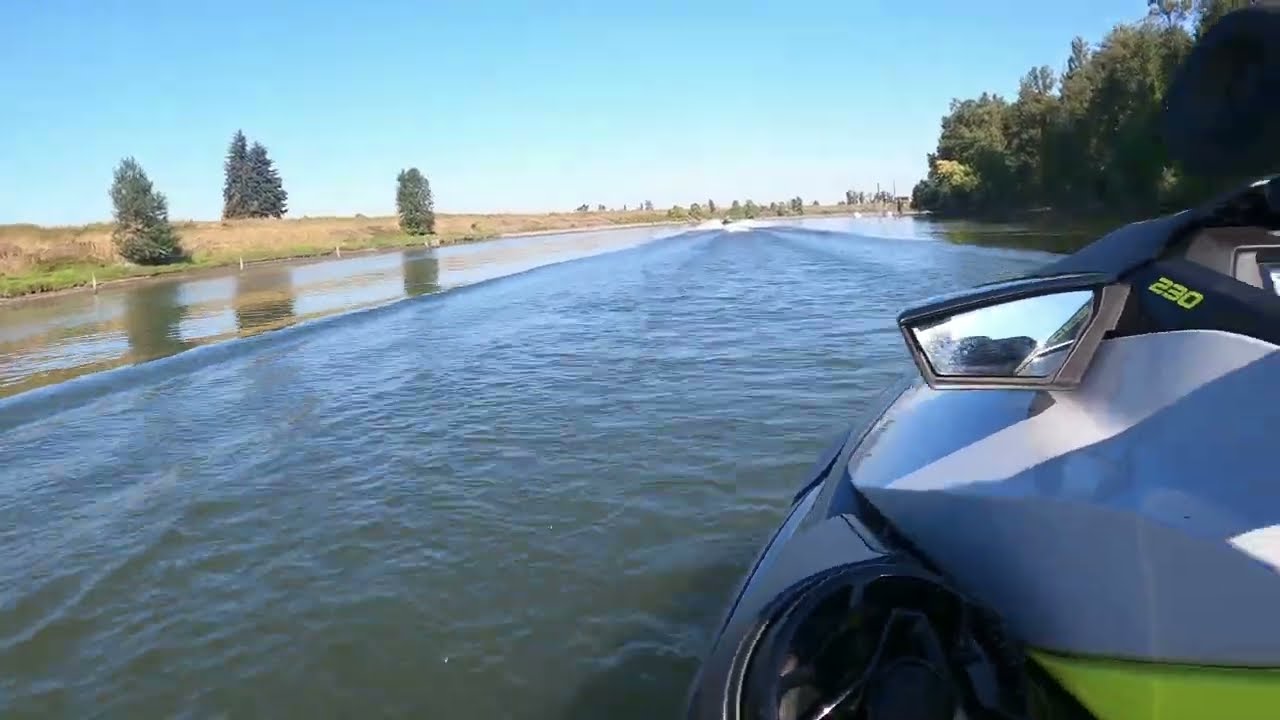This detailed photograph captures a vibrant, cloud-free sunny day on an inland body of water, possibly a lake, channel, or river. The viewer's perspective is from the side of a dark green, dark blue, and light green jet ski, prominently positioned on the right-hand side of the image. This jet ski features the number "230" in lime green, slanted characters, and includes a roughly rectangular rearview mirror. The water below is a bluish-green color, and it shows significant ripples and waves.

In the upper part of the image, dense forests with countless trees are visible to the right, while the left side shows fewer trees, some tall brown grass, and the grassy shore extending into the distance. The scene extends to another jet ski in the middle of the upper section, which creates a broad wake and white foam that disturbs the otherwise calm water. The far distance reveals buildings, enhancing the sense of depth.